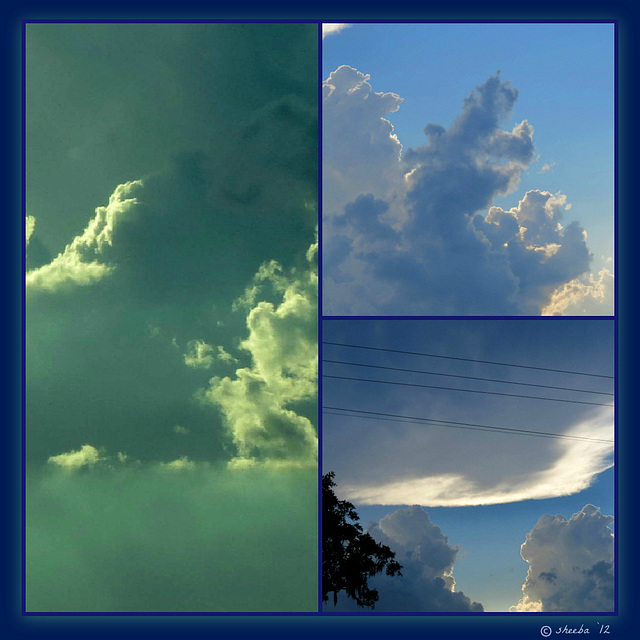This image is a square composition framed by a dark blue border, featuring three photographs of the sky. The left half of the composition contains a single rectangular image, vertically oriented, showcasing cumulus clouds tinged with a greenish-yellow filter. Sunlight illuminates parts of these clouds, casting a unique hue, possibly taken through an airplane window. The right half of the composition includes two square photographs stacked vertically. The upper image displays a bright blue sky with sunlit clouds, where the sunlight highlights the right edges of the cloud formations. The lower image appears to capture the sky from ground level, distinguished by thick cloud cover illuminated from underneath by the setting sun, giving them a soft white glow. Intruding slightly into this lower right photo are tree branches on the left and power lines crossing the top. The entire piece is subtly credited with a small copyright mark in a scripted font, potentially reading "Shida '72."